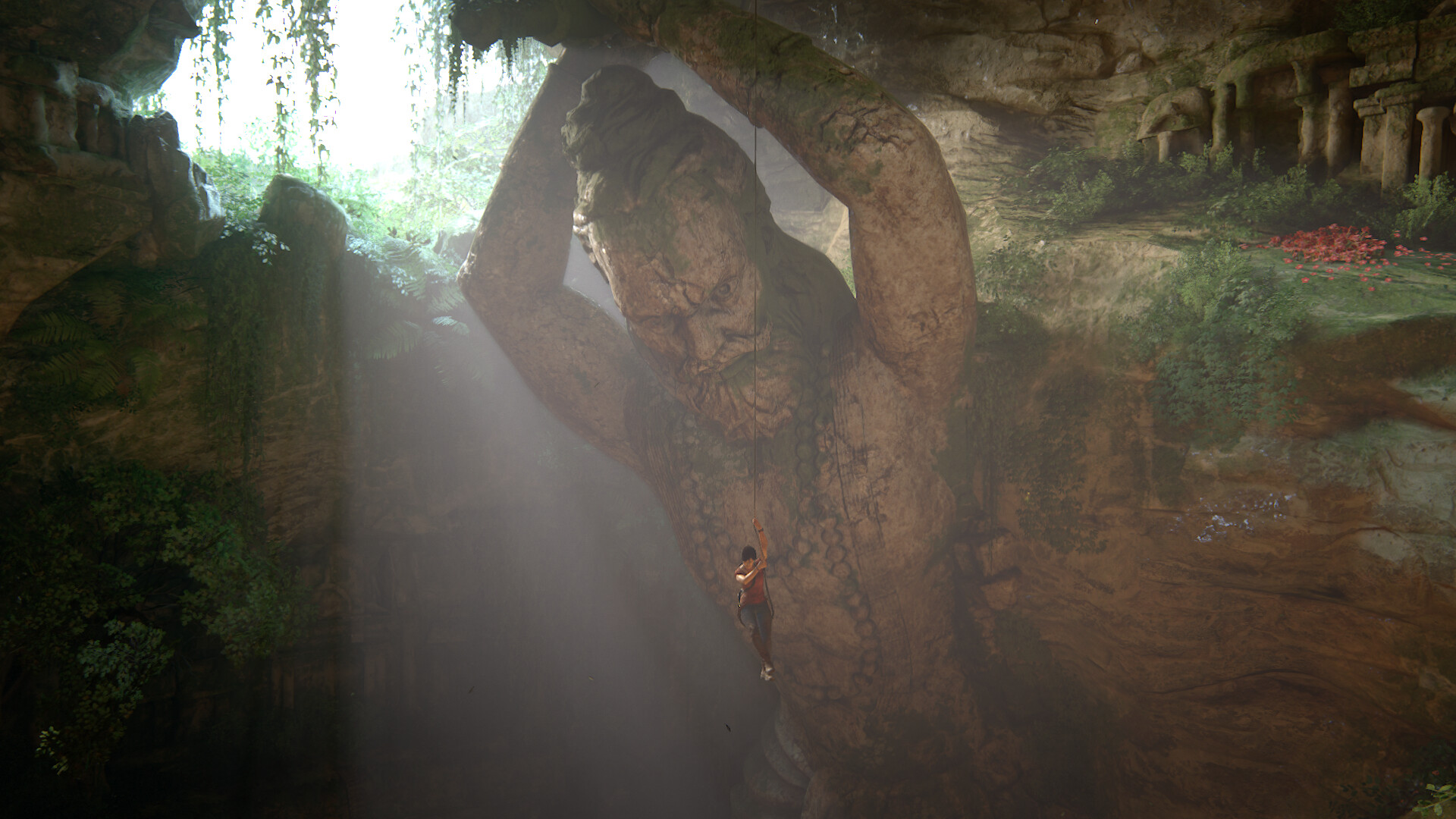This image captures a striking scene that blends natural and artistic beauty. Set within a canyon adorned with rugged rocks, the environment is cast into deep shadows, save for an opening that bathes the scene in a radiant beam of sunlight. From the rocky cliff emerges a colossal stone figure that looks like a samurai, chiseled with remarkable detail. The stone samurai stands with his muscular arms raised overhead, revealing a bare chest, a coiled topknot of hair, a heavy beard, and a fierce expression. Adding a dynamic element to the stillness of the stone, a human figure dressed in a short-sleeve red t-shirt, long pants, and sturdy shoes is rappelling down from the samurai's elevated stone arm. Their dark hair flows freely as they are suspended mid-air, gripping the rope with precision and skill. The interplay of light and shadow, combined with the grandiose sculpture and the intrepid climber, creates an awe-inspiring and adventurous tableau.